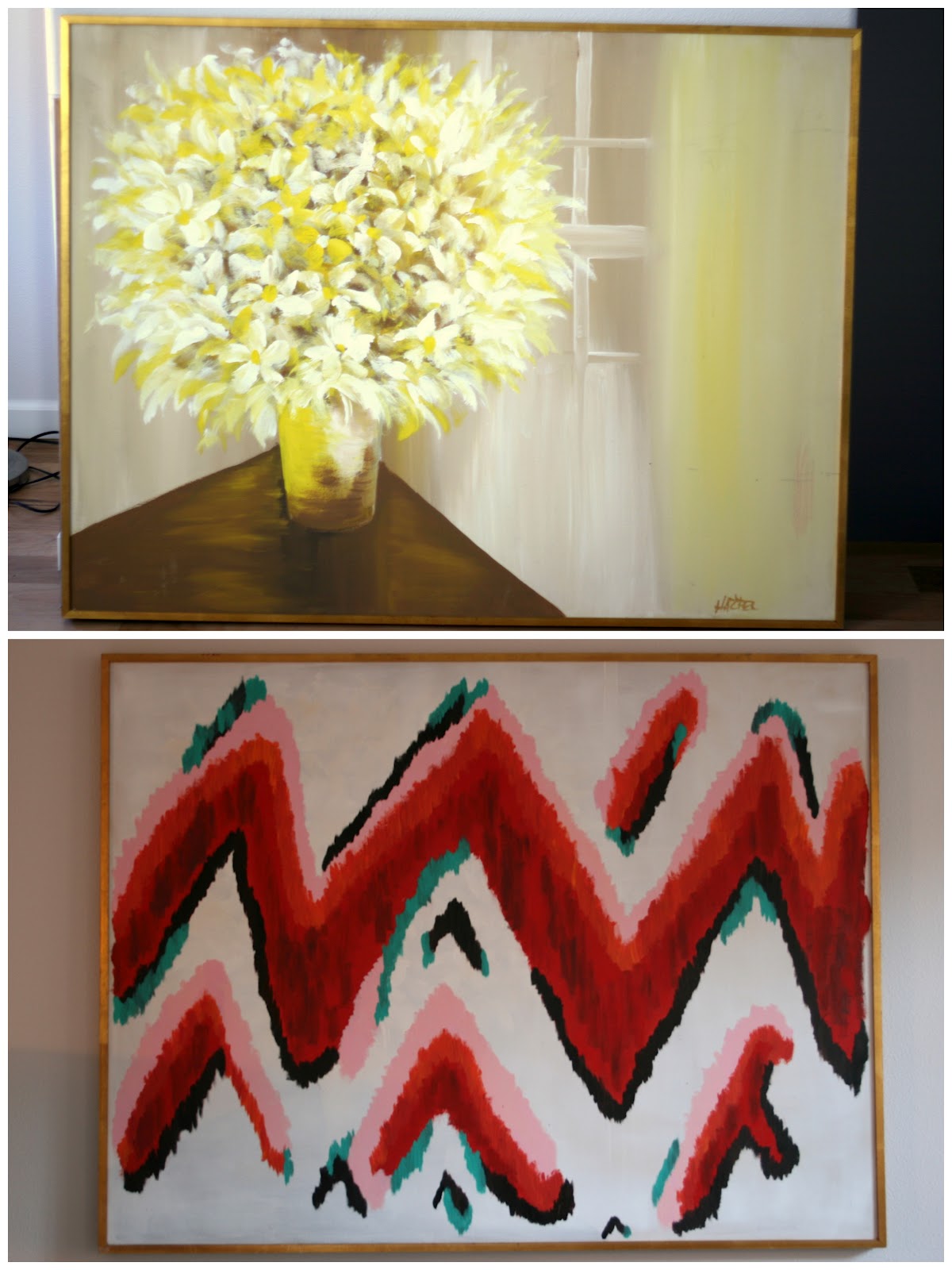The composite image features two distinct paintings, each enclosed in a thin gold frame and aligned vertically. The top painting appears to be a watercolor of a corner setting with a hardwood floor and white trim molding. The focal point is a yellow and brown vase holding daisy-like flowers in yellow and white, set against a backdrop of white walls with a window framed in white trim. The right portion of the painting showcases a wall with soft yellow streaks. The entire piece has an airy, light ambiance, suggesting a serene and simple interior space. There's a signature at the bottom, adding an element of authenticity but it's too small to read clearly.

The bottom painting exudes a modernistic style with bold horizontal zigzags resembling chevrons. Dominated by thick red lines, the zigzag pattern is accented by a lining of pink, black, and small touches of teal. Underneath the prominent zigzag stripes are smaller chevron shapes in varying red and pink hues, outlined by blue borders that provide structure and depth. This modern artwork is set against a light beige or off-white wall, contrasting the more classic, serene subject above.